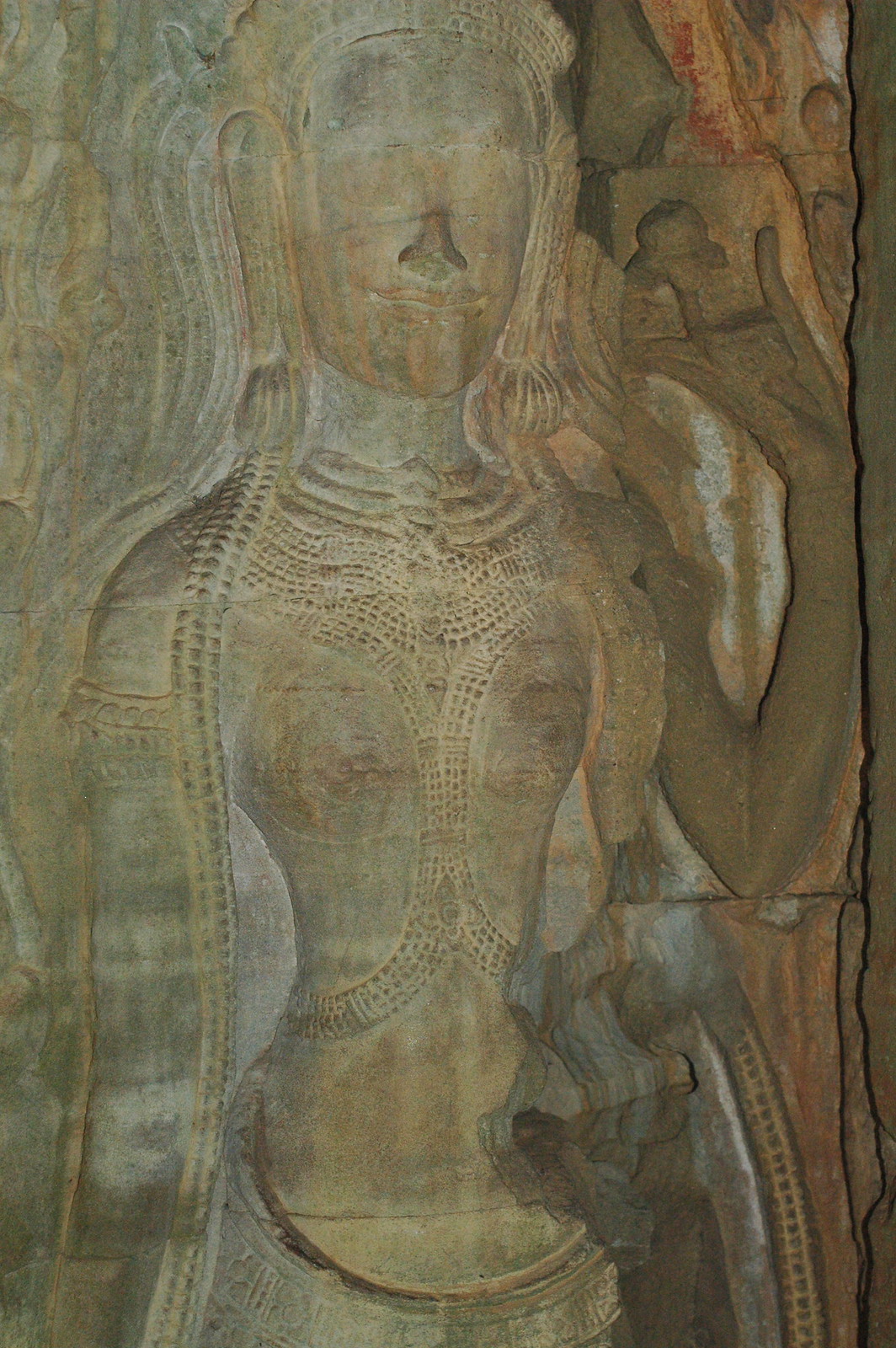This image appears to be a close-up of a weathered and intricate painting. The predominant colors are a range of tans and beiges, which are interspersed with swirls of gray and blue, giving the impression of a textured stone surface. At the center of the painting is the faint, ethereal shape of a person with their eyes closed. This figure has a prominent nose and subtly smiling lips, exuding a sense of calm and contemplation. Bands, possibly bracelets or armlets, are visible on one of the figure’s arms, adding a touch of detail to their otherwise soft appearance. The figure exhibits a notably slim waist, enhancing the delicate nature of the portrayal.

The painting’s edges are notably frayed, appearing weathered and tattered, which suggests either age or an intentional artistic choice to convey a sense of antiquity. The right side of the painting is characterized by darker browns mixed with lighter blues, creating a rich contrast that adds depth to the overall composition. The careful arrangement of colors and the detailed depiction of the central figure make this painting a compelling and evocative piece of art.